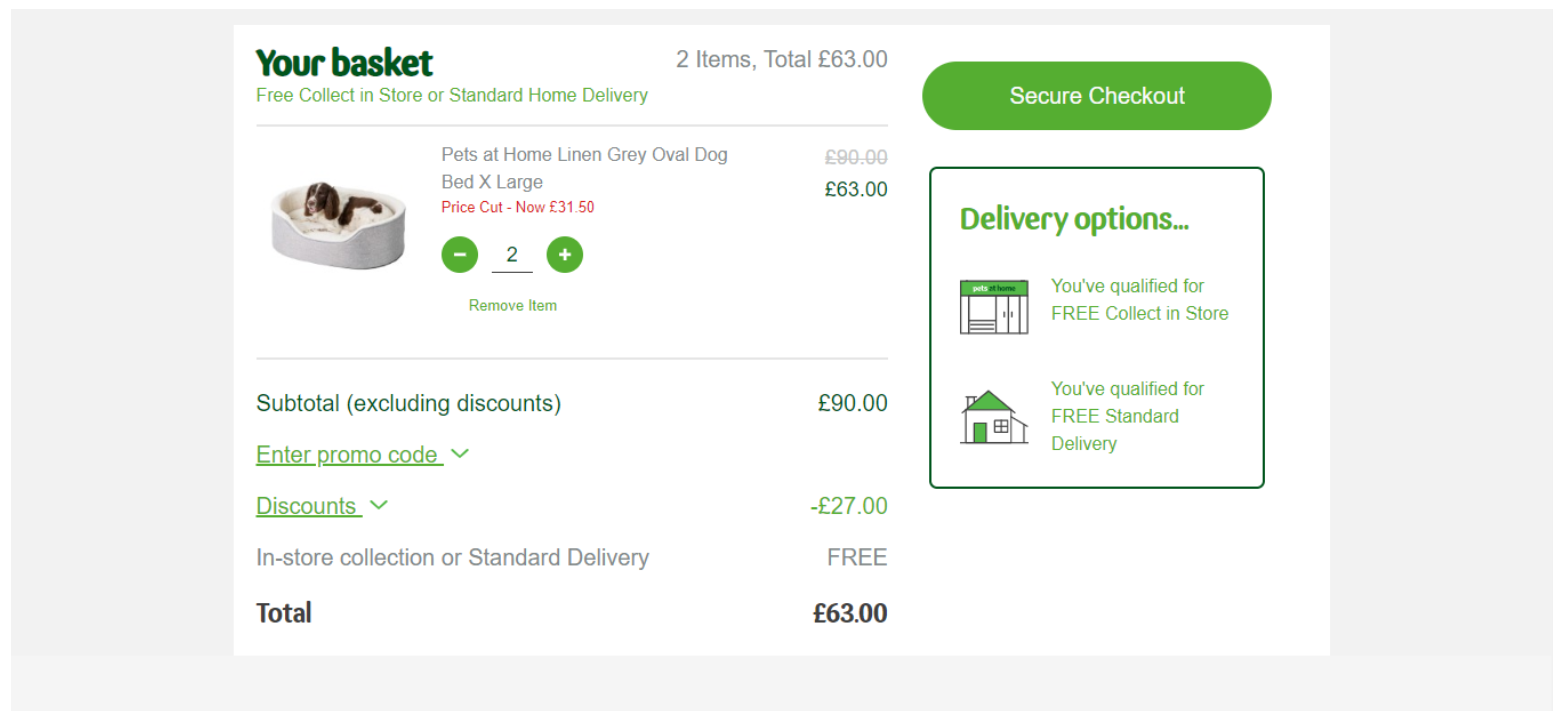The image depicts an online shopping page from a pet store. At the top, the text "New Basket" is prominently displayed. Below this, a summary reads: "Two items, total: $63." There's an option bar with "secure checkout" highlighted in green.

The page features an image of a puppy nestled in a gray, linen oval dog bed from the "Certain Pets at Home" collection. The bed is marked as size XL and has a price cut to $31.50. There's functionality to adjust the quantity of this item using plus and minus signs, as well as an option to remove the item.

At the bottom, there's a subtotal excluding the discount amount, indicated to be $90. A $27 discount is applied, resulting in the final total of $63. There's also an option to enter a promo code.

On the right side of the page, under "Delivery options," it notes that the purchaser has qualified for both free collection and free standard delivery.